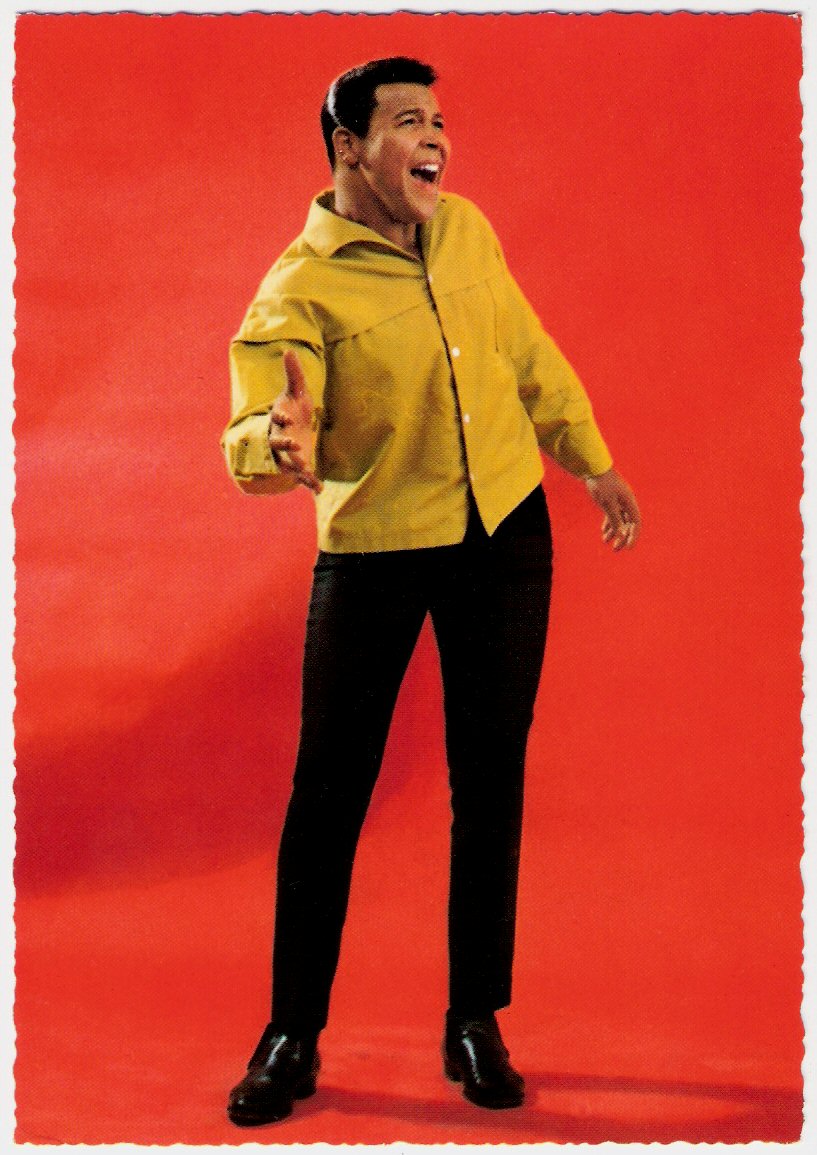The image depicts a young African American man from perhaps the 1950s or 60s, captured in a professional photo shoot against a solid red backdrop. He is dressed in a loose, mustard-yellow, long-sleeve shirt with a collar, paired with black pants and shiny black high-heeled shoes. His short, wavy dark hair frames his smiling face, with his mouth wide open in a joyous expression, revealing big cheeks. He is slightly bent at the waist, with his right arm bent and held in front of him, while his left arm is extended behind. The man appears to be singing, facilitated by a headset with a microphone around his head. The image has a scanned border, emphasizing the retro aesthetic of the photograph.